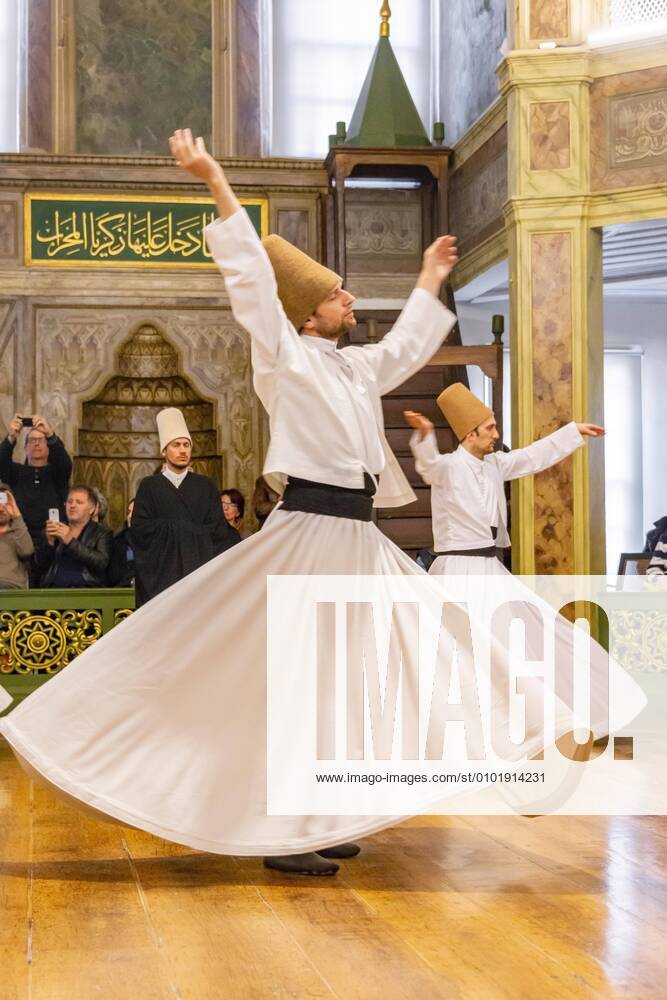This image captures a vibrant scene of two men dancing on a brown hardwood floor, donned in traditional Middle Eastern attire. They are clothed in long white robes with matching sashes and long skirts, and they are wearing tall, square, thimble-like brown hats. Their shoes are a dull, dark brown felt. Behind them are onlookers eagerly capturing the moment with their cameras. There is another man standing in the background, also adorned in traditional attire: a long black cape and a similarly tall but lighter brown hat. The backdrop features intricate stone walls with arches, decorated with gold filigree and a green panel showcasing golden Islamic calligraphy. Overlaid on the image is a white box labeled "imago" with the text "www.imago-images.com/st/0101914231" in black underneath.